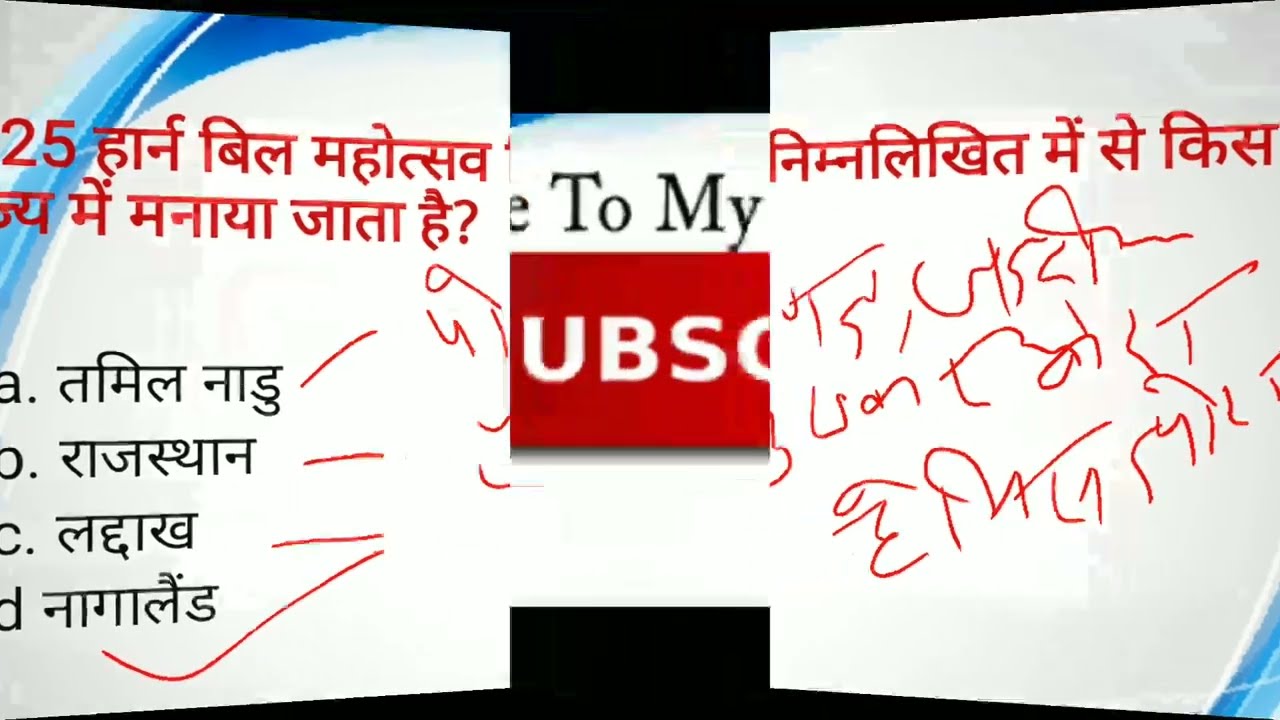This image depicts a collage of textual content, primarily featuring writings in a foreign script that appears to be an Asian language, possibly Arabic or Indian, characterized by connected characters through a straight line at the top. On the left side of the collage, a smaller poster showcases text in red and black with a decorative wave gradient in blue at the top. The right side mirrors this, containing similar text, albeit with a less elaborate background featuring a small segment of the blue wave at the bottom right. The background for the entire collage is predominantly black, although it is mostly obscured by the various elements. Centrally positioned, some English words are visible, with the readable phrase "to my" in black, accompanied by a red box with white, capital letters stating "UBS." Additionally, numbers and bullet points starting with A, B, C, and D are evident on the left side, contributing to the overall impression of a presentation slide, possibly created using PowerPoint or a similar medium. Hand-drawn squiggles in red pen accentuate parts of the text, enhancing the collage's artistic and informal presentation style. The color palette primarily includes shades of gray, light blue, dark blue, red, black, and white.